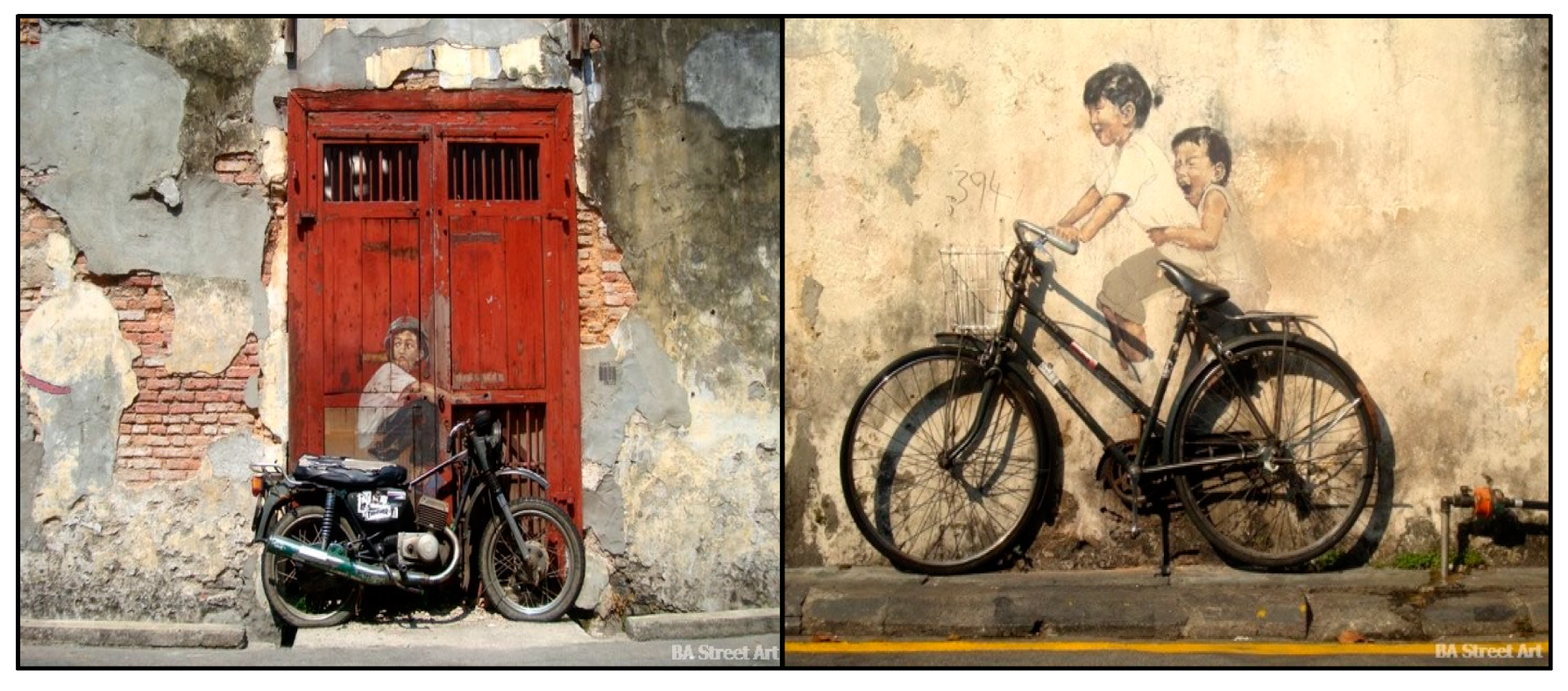The image features two pieces of street art side by side, divided by a thin black line, each encapsulating an imaginative blend of reality and painting. On the left, there’s a deteriorating cement wall revealing the red bricks underneath, with an aged red double door at its center. This door has grates or bars on the top and bottom of each window and in front of it is parked a realistic black motorcycle accented with silver. Painted on the door is a figure, cleverly positioned to appear as if riding the real motorcycle. The scene, set on a concrete street, has a gritty urban charm. On the right, against a similarly worn cement wall with hues of gray, two young figures with dark hair are painted to look as though they are riding a real adult-sized bicycle leaned against the wall. Both artworks are marked with "B.A. Street Art" in the lower right-hand corner, merging the tangible objects with the painted ones to create lively, interactive street scenes.